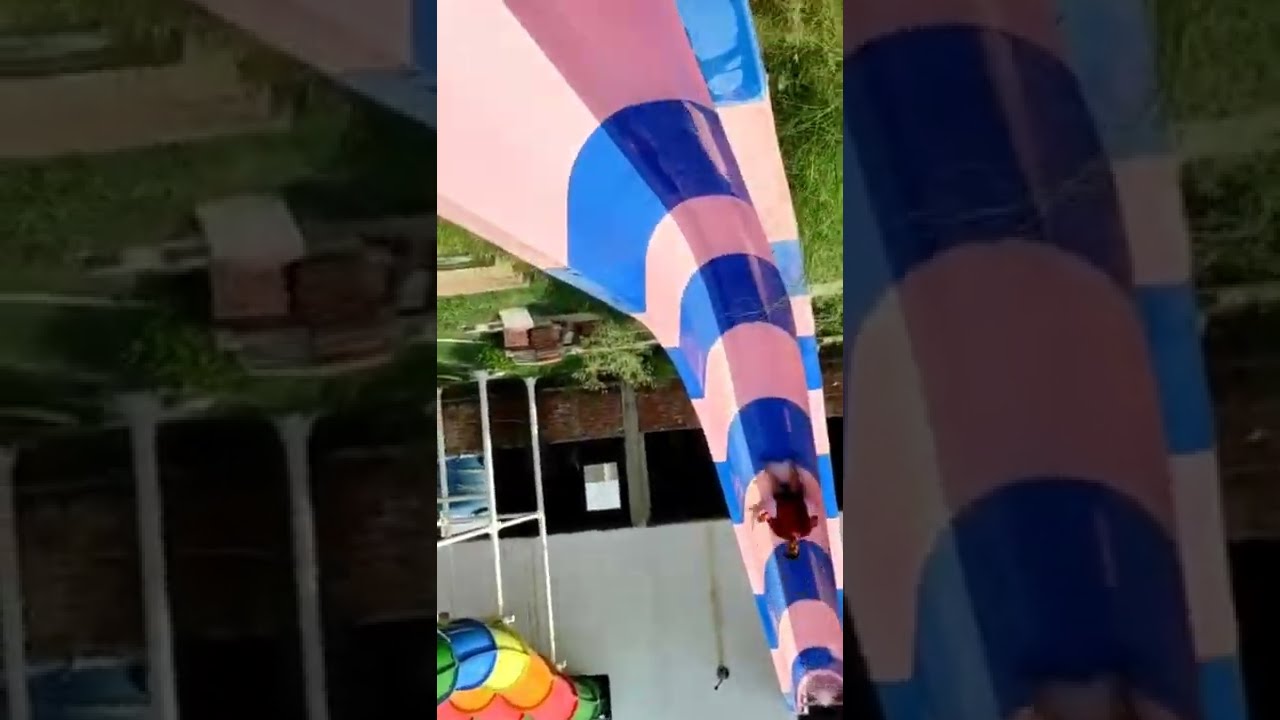The image appears to be a flipped screenshot of a social media post, possibly from Instagram or TikTok, taken during daytime at an outdoor or partially abandoned water park. Dominating the scene is a long, narrow, pink and blue striped slide. Amidst a green grassy area, a person dressed in a red bathing suit or shirt and shorts is descending the slide. The background features an enlarged portion of the main image showing more of the surroundings. Behind the slide, a white wall, possibly rust-streaked where water may have once flowed, is visible along with a tall white iron shelf. Also noticeable in the upper right corner is a colorful rainbow object featuring green, pink, orange, yellow, and blue hues. The lower left-hand side reveals another slide or structure, contributing to a sense of an intricate water park layout that may have seen better days.